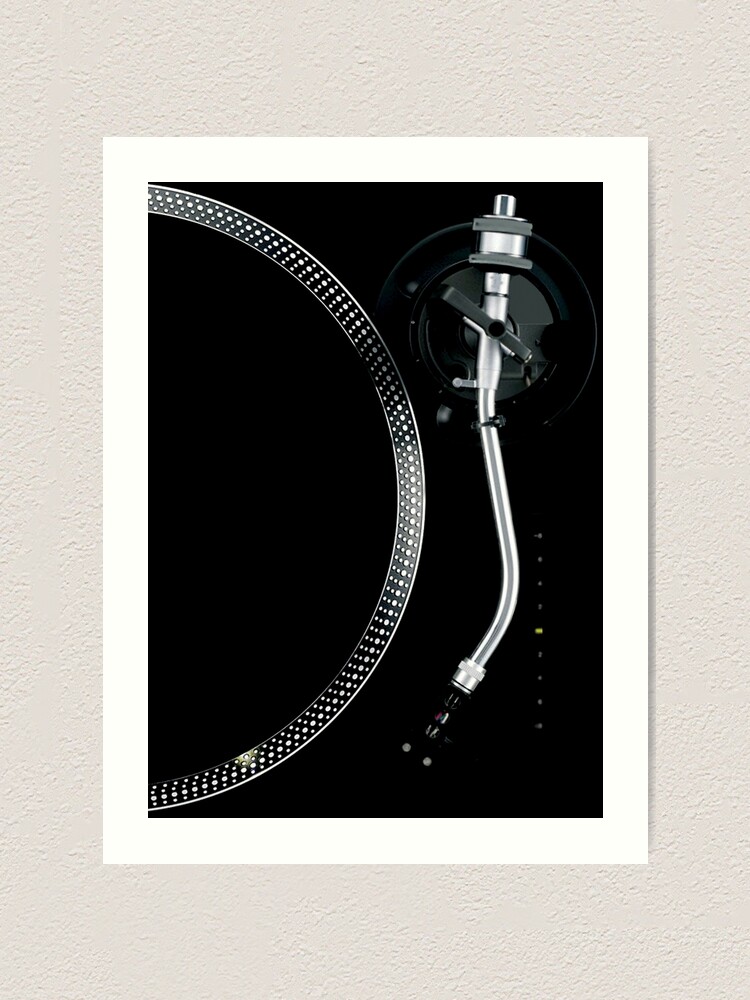A black and white photograph is positioned on a light gray sheet of paper. The photograph features a close-up of an old-fashioned record player, showcasing a large, round turntable made of silver-colored metal. The turntable surface is dotted with small, raised bumps, resembling tiny brads. Adjacent to the turntable is a long metallic tonearm, which is silver with a black tip. The back end of the tonearm is supported by a black plastic mechanism that enables its movement. At the front, the black tip houses the needle that rests on the record. To the side are several buttons that control the volume and other functions of the record player. The contrast in the photo starkly highlights the intricate details of the vintage audio equipment.